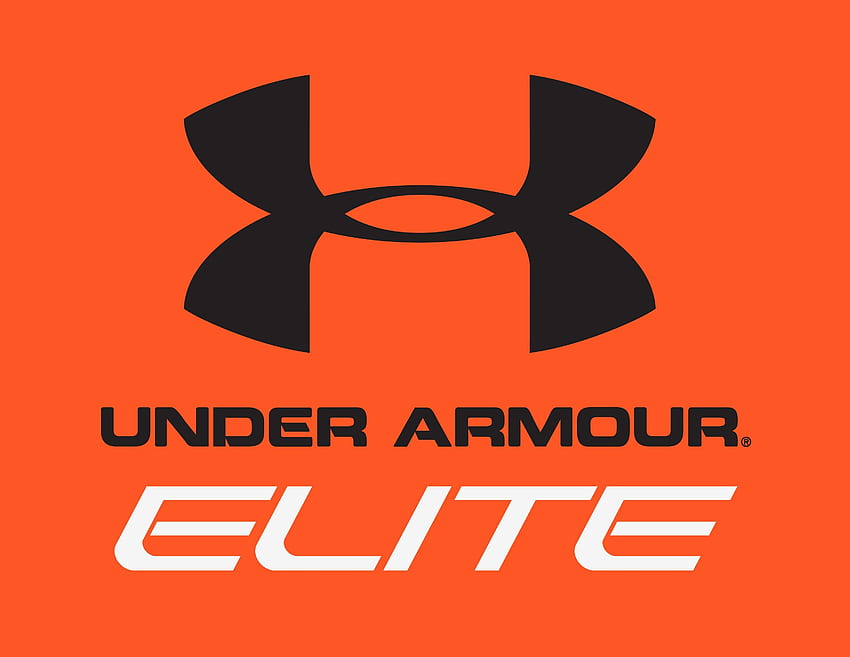The image features a centrally positioned Under Armour logo in black against a bright orange background. Directly beneath the logo, the brand name "Under Armour" is written in bold black text. Below this, the word "Elite" is prominently displayed in larger black letters. A trademark symbol appears beside the "Under Armour" text, affirming the logo's authenticity. The composition is striking with its limited color palette of orange, black, and white, effectively highlighting the brand's new elite offering.